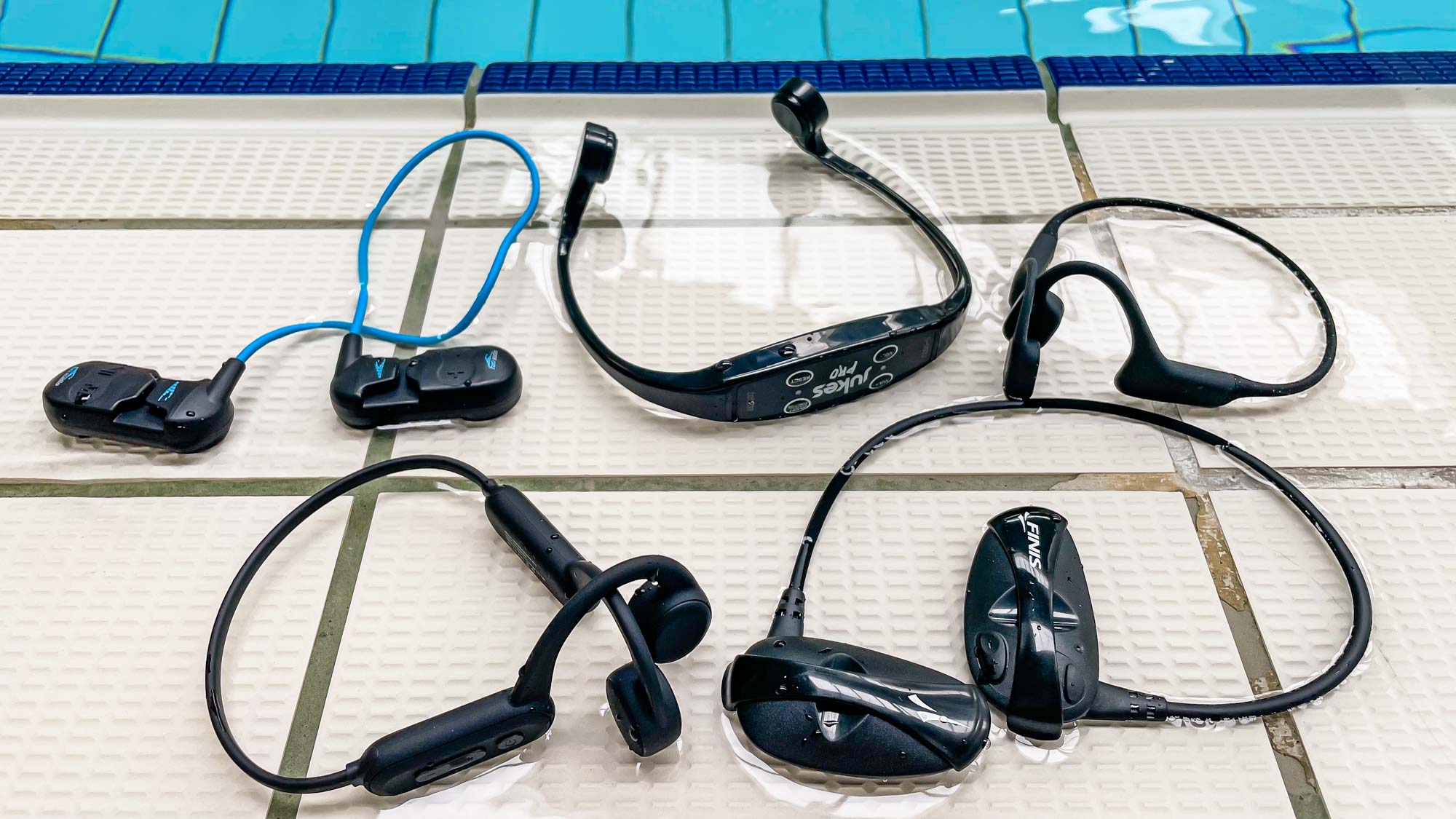This image is a detailed color photograph of the edge of an indoor swimming pool, showcasing a wet tiled surface dominated by white tiles with some light blue water visible along the top edge. Positioned on these wet tiles are several black electronic devices, likely waterproof earbuds designed for use while swimming. 

At the top left, two cylinder-shaped capsules are connected by a blue cable, and nearby, there's a black semicircular device featuring a central panel. On the top right, a C-shaped item appears to be earphones designed to go around the back of the head. Another set of similar C-shaped earphones rests at the bottom left, each ending with rounded circles. Lastly, the bottom right device, labeled with white text "FINIS," consists of two capsule-shaped ovals connected by a black cable. The wet surface of the tiles emphasizes the aquatic environment these devices are intended for.